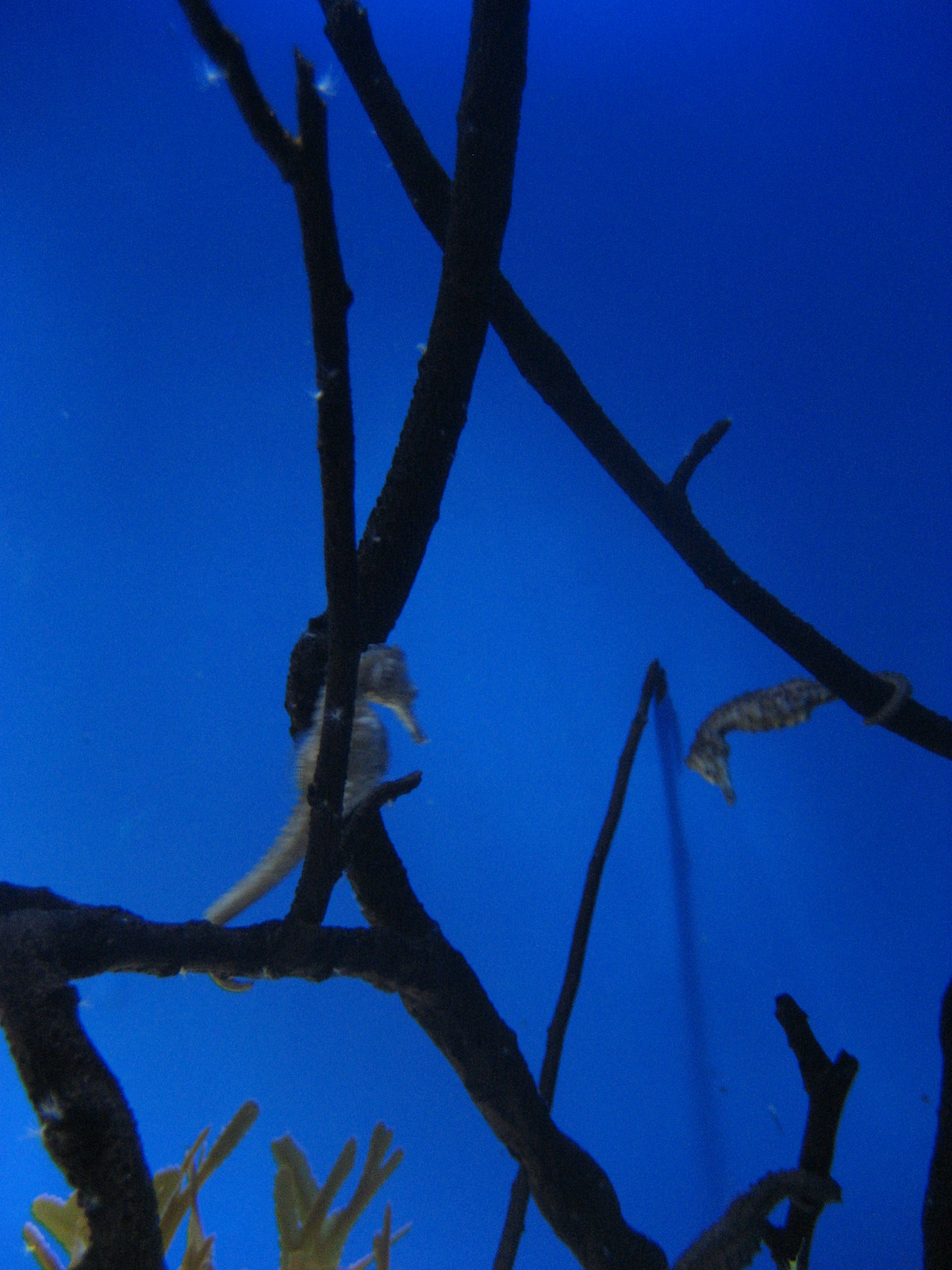The image captures an aquarium scene with deep cobalt or royal blue water, creating an ethereal, night-sky-like backdrop. Twigs or branches, appearing black, spread intricately throughout the frame. Toward the bottom, yellowish seagrass or a fern-like plant adds a touch of contrasting color. Two small seahorses are present in the image: one on the right with its tail wrapped around a branch, its semi-translucent, yellowish body extending horizontally towards the left. The second seahorse, positioned centrally, is more visible and light-colored, with its tail slightly curled around a horizontal branch; however, its body is partially obscured by vertical branches. Pinpoints of light twinkle around the branches, adding to the otherworldly effect. The aquarium itself is rectangular, approximately six inches tall and four inches wide, with a distinct shadow cast on the background, revealing it's set against a wall.